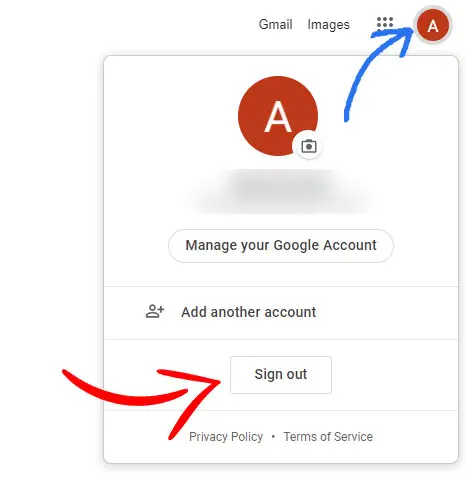Detailed Caption:

The screenshot showcases a mobile device with a white background. On the right-hand side, there are several elements. Firstly, there are familiar Gmail icons, followed by a cluster of six gray dots arranged in a 3x3 grid, although the bottom three dots are obscured by a blue horizontal line. Next to this, a gray circle contains a smaller brown circle featuring a white 'A' in the center. A crudely drawn blue arrow appears to be pointing at the 'A'.

In the center of the image, another white box displays a similar 'A' mechanism. Toward the bottom right of this box, there's a smaller gray circle intersecting with a gray camera icon. Another section of the screenshot is blurred out, possibly to hide sensitive information.

Two primary buttons are positioned below: one black button labeled "Manage your Google account," and another button featuring a person icon with a checkmark, labeled "Add another account." Directly below these buttons, the option to "Sign out" is available, marked by a prominent, neatly drawn red arrow.

Finally, at the bottom center of the screenshot, there's text in gray reading, "Privacy Policy" and "Terms of Service." The image is devoid of any additional elements or annotations.

Note: The last few lines of the provided text reflect a personal message and are omitted from this detailed caption.